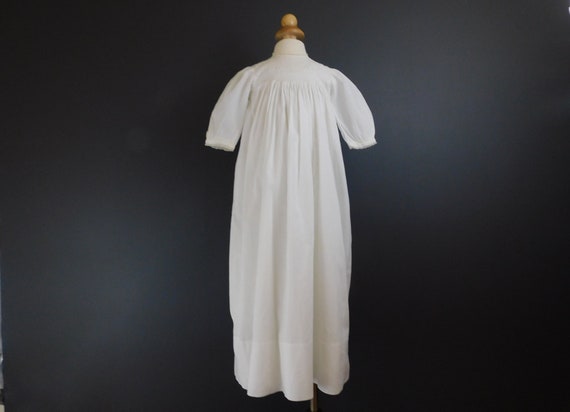In the center of this photograph with a gradated black background, stands an old, white nightgown, hanging on a wooden hanger or possibly a stand designed to display garments. The background transitions from deep black in the corners to a slightly lighter gray towards the middle, providing a subtle contrast to the garment itself. The gown, which reaches down to the floor, features short sleeves and a loose, flowing fit. There's pleating detail that starts at the chest and continues down the fabric, creating gentle waves towards the bottom. The nightgown, reminiscent of the 1800s era, evokes a time when lighting candles was a nightly routine. This simple yet evocative image captures the essence of a bygone era with the gown’s modest, unembellished elegance.